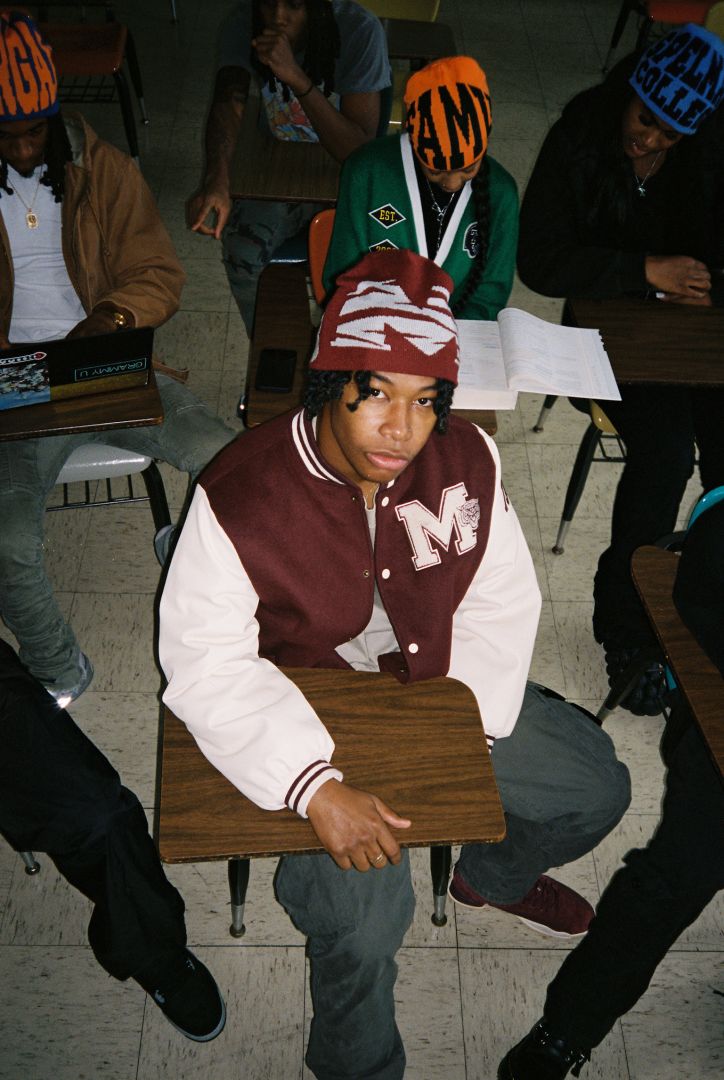This photo captures a young African American male seated in a classroom, taken from an overhead perspective, focusing on him among a group of students. He is donning a maroon and white letterman jacket with a prominent white 'M' on the left chest and matching maroon and white beanie, also displaying the letter 'M.' He appears pensive, gazing up at the camera with his right arm extended across the brown, wooden desk, gripping its edge. His attire includes bluish-gray pants and dark maroon sneakers. The classroom setup includes rows of similar brown wooden desks with black metal legs featuring silver feet. Behind him, three other students are visible. The student to his left is wearing a brownish jacket and a beanie that seems to say “Bengals.” To his right, one student wears a green jacket and a green beanie, focused on a book open before them, and another student is dressed entirely in black with a blue beanie. These students appear engrossed in their studies, contributing to the academic atmosphere of the setting.